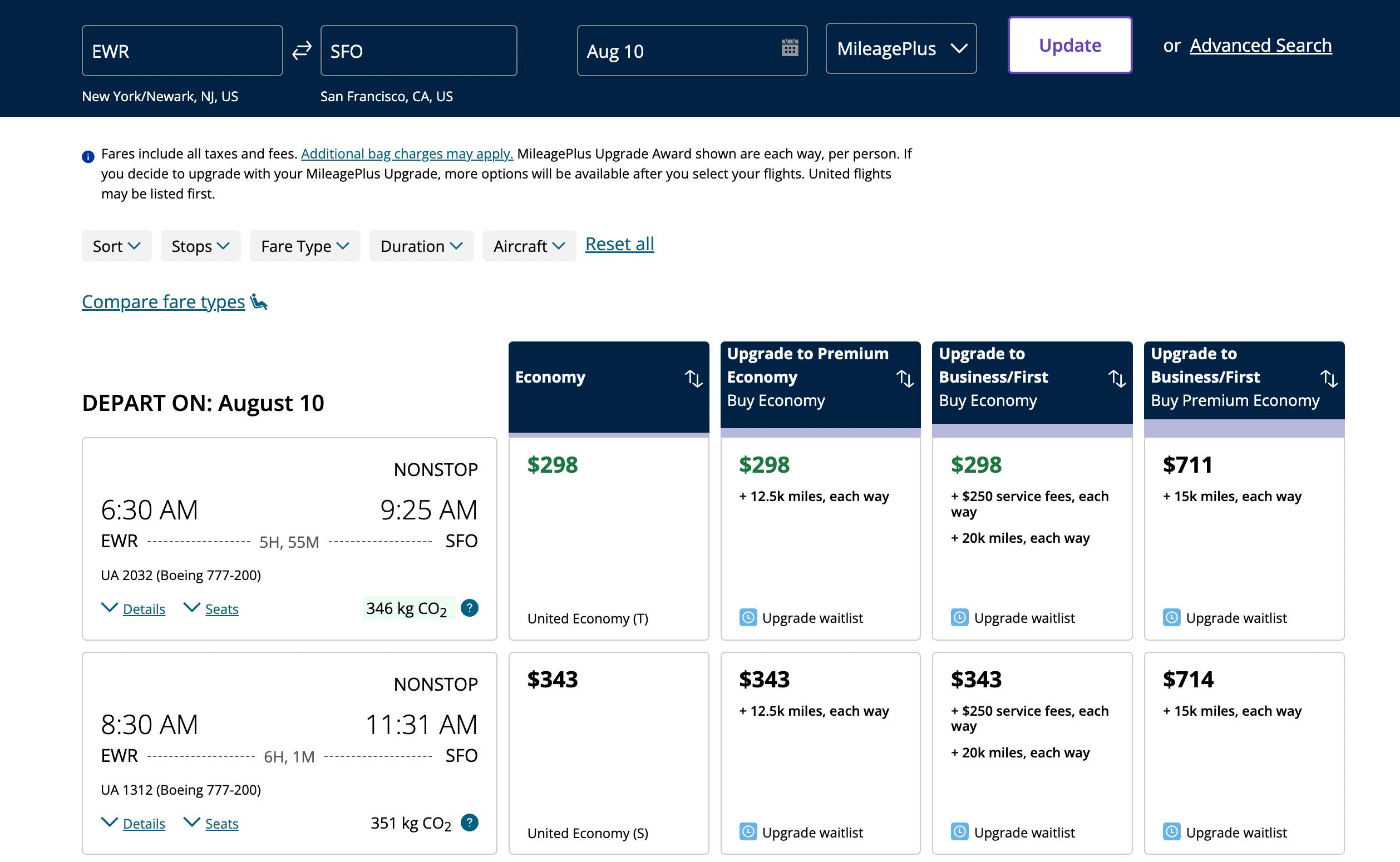The image displays a detailed flight booking interface. In the top left corner, the departing and destination airports are shown: EWR (Newark, New Jersey, USA) to SFO (San Francisco, California, USA), with a departure date of August 10th. There are interactive elements such as the "MileagePlus" dropdown and an "Update" button in white. Additionally, an "Advanced Search" option is available in the top right corner of the screen.

Beneath these, a notice indicates that fares include all taxes and fees, with additional charges for baggage possibly applicable. MileagePlus upgrade awards are specified as one-way per person, and more upgrade options will appear after flight selection. United flights are likely listed first.

The interface contains various dropdown filters labeled "Sort," "Stops," "Fare Type," "Duration," and "Aircraft," along with a "Reset All" link. There is also an option to "Compare Fare Types."

Following this, the schedule for August 10th is shown, listing two non-stop flights from Newark to San Francisco. The first flight offers the following fares:
- Economy: $298
- Premium Economy: $298
- Business/First Class: $298
- Business/First Class (upgraded from Premium Economy): $711

The second non-stop flight departs at 8:30 AM and arrives at 11:30 AM. The fares are:
- Economy: $343
- Premium Economy: $343
- Business Class: $343
- First Class: $714